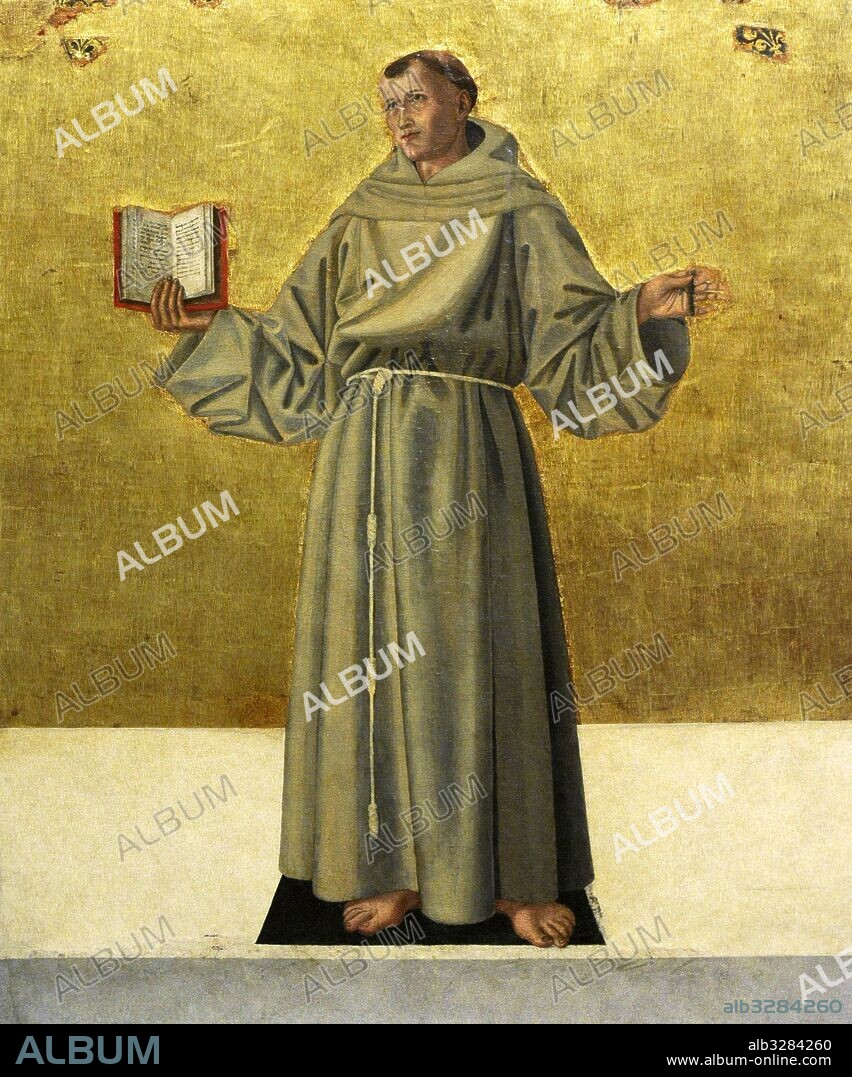The image depicts an ancient painting of a religious figure, likely a saint, standing barefoot in a long, greenish-brown robe with a white rope cinched around the waist. The saint has a book open in his right hand, presumed to be a Bible, revealing both pages. His left hand appears to hold a corkscrew-like object. The background from his knees up is gold, transitioning to a cream-colored floor below, with a gray band at the bottom resembling a pedestal. He stands on a black rectangular mat placed on a white stone surface. The image is overlaid with several diagonal watermarks repeating the text "album-online.com" and includes an identifier, ALB3284260, at the bottom right.